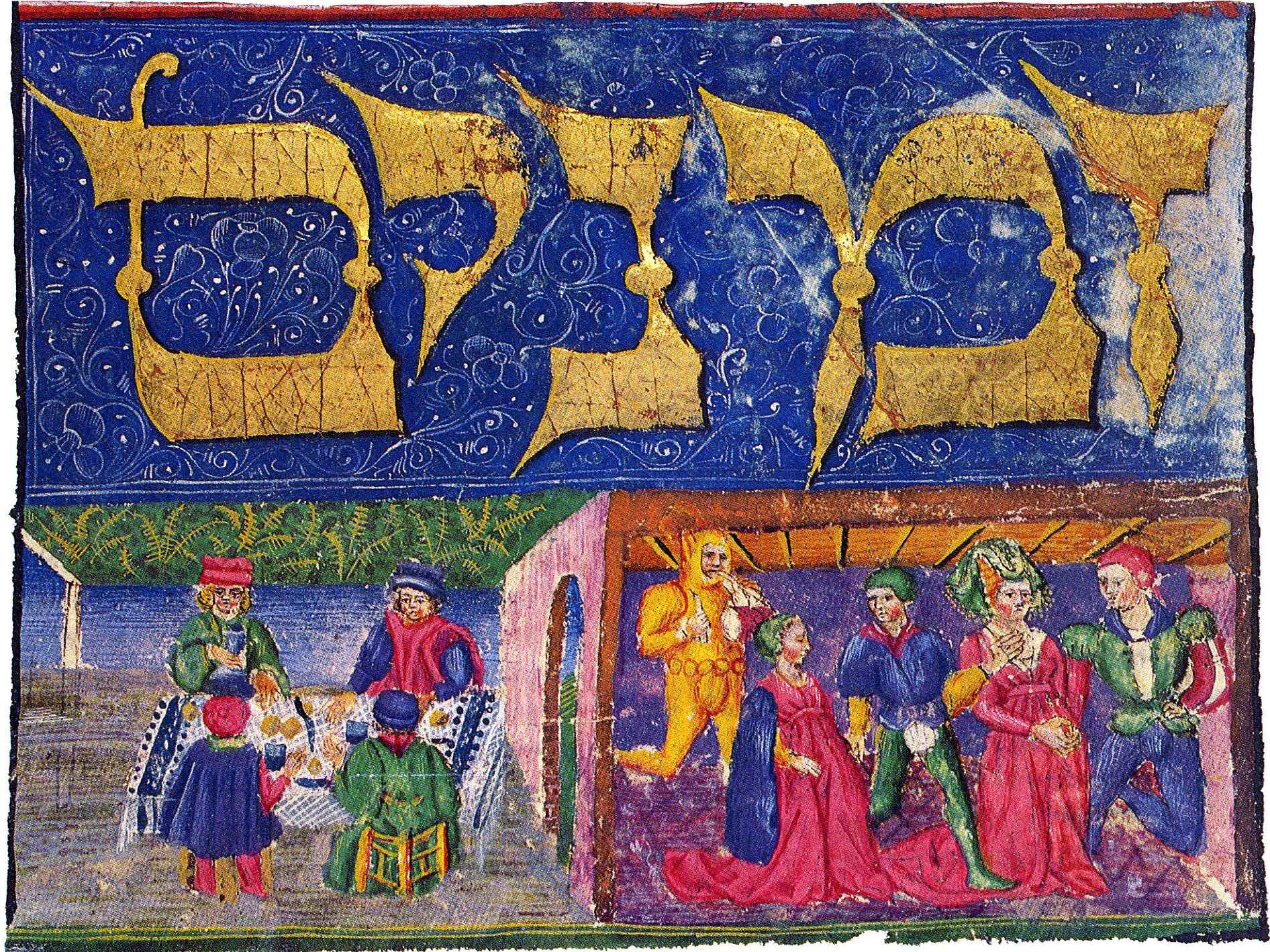The image depicts a detailed medieval painting with distinct sections. At the top, there's a horizontal rectangular panel featuring gold Hebrew letters set against a deep navy blue background adorned with intricate white botanical and curly designs. In the lower part, the painting is divided into two scenes. 

On the right, there's an arched building. Inside the arch, several people are gathered, clad in vibrant attire: a man in a one-piece yellow suit, two women in long pink dresses, and two men in blue and green garments. They appear to be engaged in a social gathering. 

Outside the building, to the left, there is a rectangular table covered with a white and blue tablecloth. Four people are seated around it, wearing similarly bright clothes (blue, pink, and green). The table is laden with bread, cheese, and a knife, suggesting a shared meal. The background is filled with more botanical designs, integrating into the scene's medieval aesthetic.